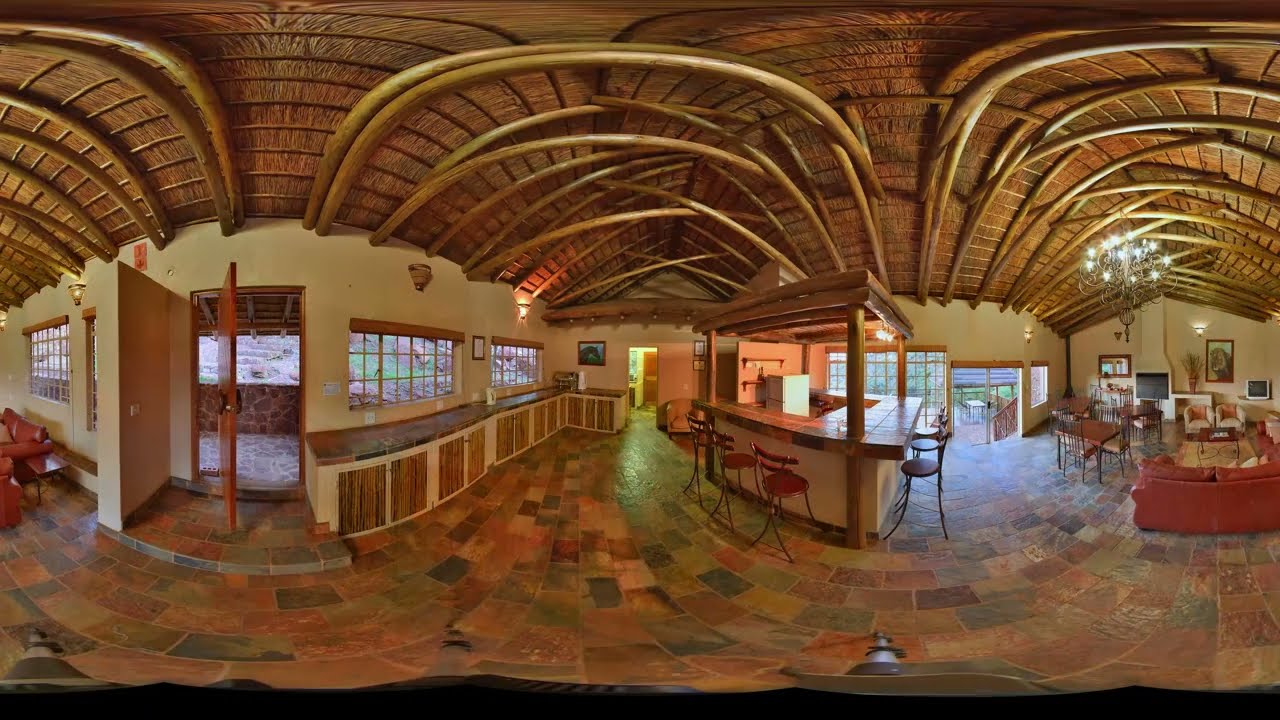The image depicts a beautifully scenic river valley, captured with a 360-degree lens, giving it a distorted, VR-like quality. The scene is centered around a charming, possibly European rooftop apartment that appears somewhat warped due to the lens. The left portion of the image features a red brick building with an open sliding glass door leading to a cozy living room furnished with two white chairs and an illuminating lamp. A piece of artwork depicting a horse's head adorns the rear wall. Moving toward the right, the image reveals a wooden deck with a railing, patio furniture including a bench, a chair, and a table, all positioned to take in the stunning valley view. The valley itself is lush with green vegetation and dotted with four or five houses nestled along the left ridge. The horizon stretches across the back of the valley beneath a clear blue sky, save for a few clouds near the horizon. The sun appears to be either rising or setting, casting a bright glow that adds to the serene and picturesque atmosphere. The entire scene is awash with vivid, professionally captured colors, contributing to its breathtaking and high-resolution quality.